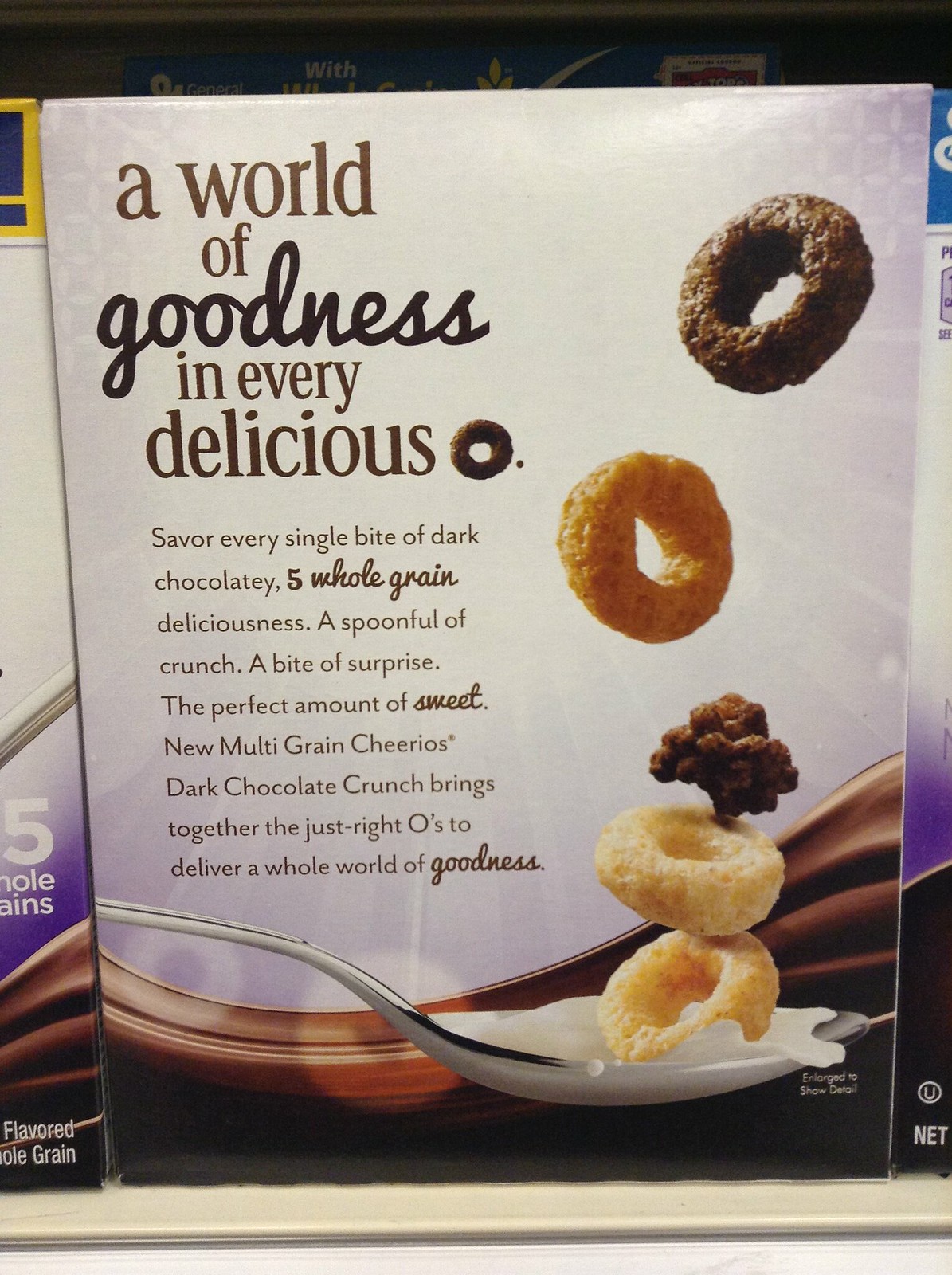This photograph captures a vibrant, green-colored shelf in a market, showcasing an array of cereal boxes. Dominating the scene is the back of one cereal box, bringing attention to its message and imagery. The box proudly proclaims, "A World of Goodness and Everything Delicious," and features an illustration of a mischievous-looking character with the tagline, "Savor Every Single Bite of Dark Chocolate." This cereal promises a spoonful of crunch and surprise, touting a perfect balance of sweetness with its dark chocolate crunch. The detailed description highlights the cereal’s beautiful appearance and the delightful combination of flavors, making it a standout on the shelf.